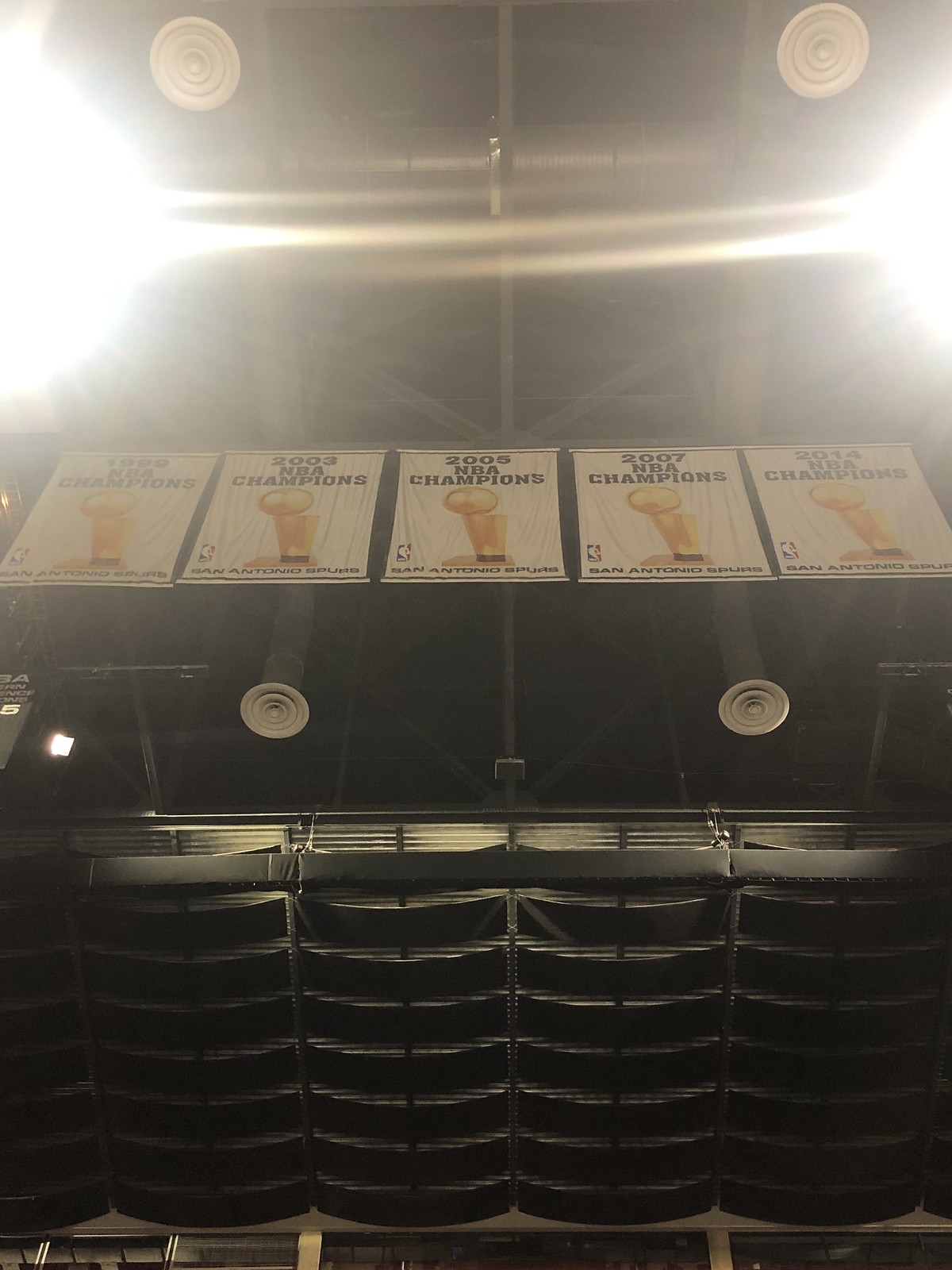The image depicts the ceiling of a sports arena, captured from the floor looking upward. Prominently displayed are five championship banners for the San Antonio Spurs, celebrating their NBA victories in 1999, 2003, 2005, 2007, and 2014. Each banner features a golden trophy icon and the corresponding year of the championship, with "NBA Champions" and "San Antonio Spurs" inscribed beneath. The banners, which vary slightly in clarity with the leftmost one being somewhat blurry, create a striking visual against the backdrop of the arena's intricate metal struts and suspended speakers. Bright spotlights at the left and right edges of the top section of the image cast an intense light, creating a slight haze that partially obscures some of the ceiling's details, including additional loudspeakers and the ceiling baffles. The overall ambiance suggests the grandeur and pride associated with the team's achievements.